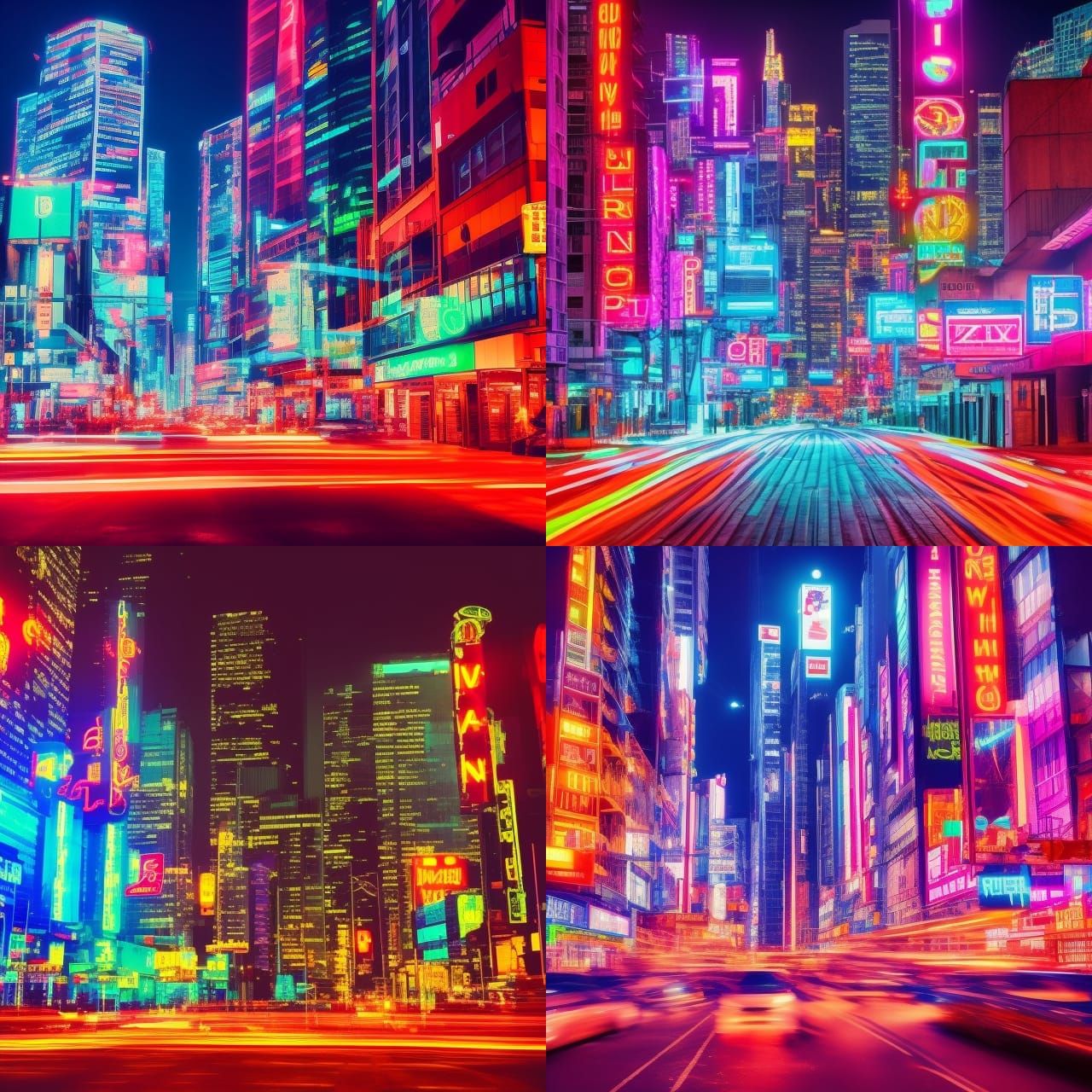A vibrant and dynamic cityscape is depicted in this photograph, divided into four distinct images, each showcasing an urban setting illuminated by a multitude of bright, neon lights. The city, which bears a striking resemblance to New York City, is bathed in a spectrum of colors, featuring buildings adorned with blue, magenta, and yellow hues. The top left image highlights predominantly blue lights in the distance, with vivid red lights in the foreground, creating a cyberpunk aesthetic. The top right image offers a street-level perspective, with motion blurs on either side and buildings lit up by pink and blue neon signs, emphasizing the city's perpetual motion and energy. The bottom left image portrays high rises with white and yellow lights, while street-level neon blue signs add a modern twist. Finally, the bottom right image captures the essence of Times Square with its motion-blurred cars and bustling street life. This lively, bustling metropolis is filled with the hustle and bustle of activity, street lights, and cars, even at night, truly embodying the vibrant spirit of an urban night scene.